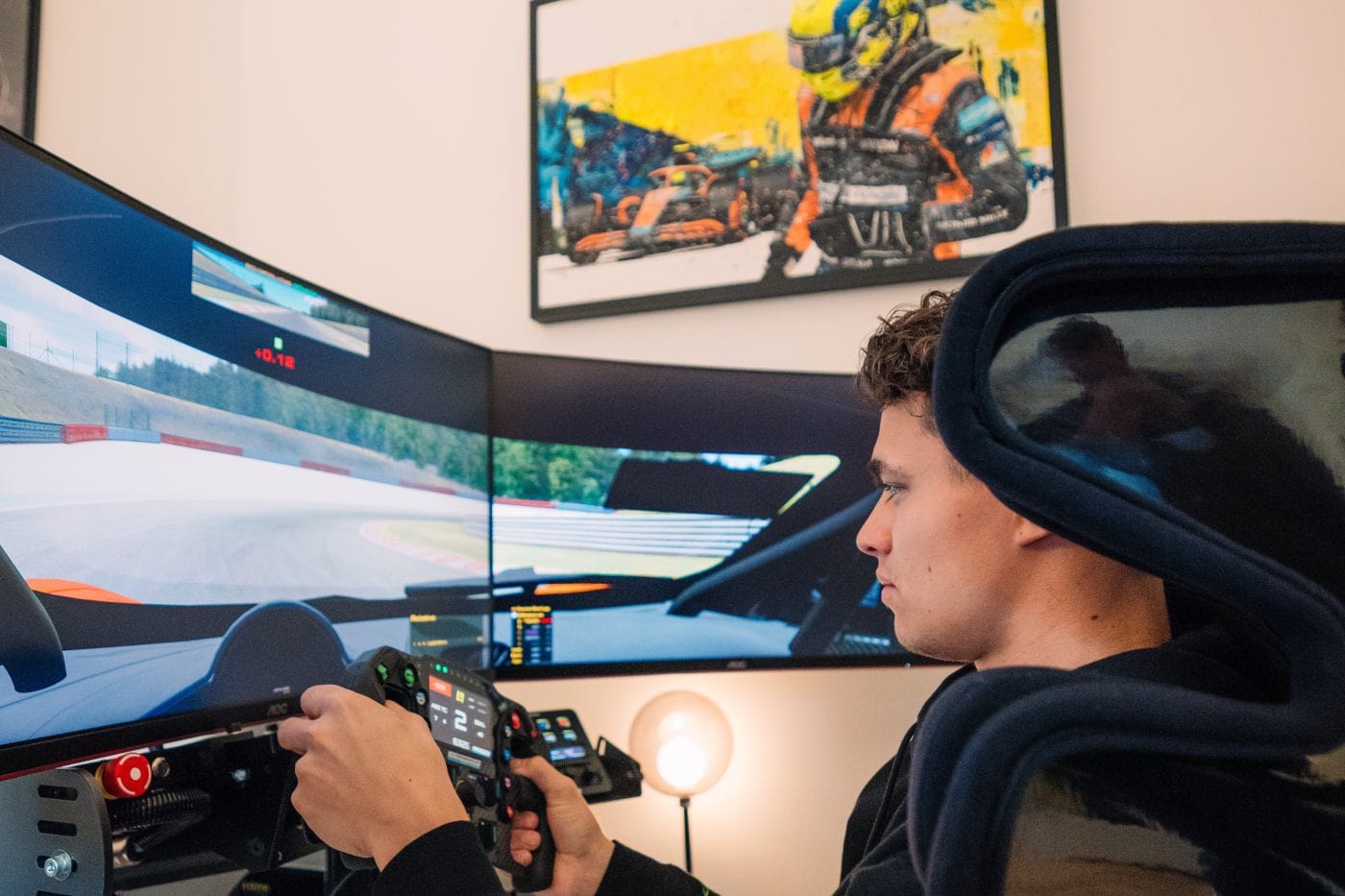The photograph depicts a young man with short curly brown hair, immersed in a sophisticated car racing simulator setup. He sits in a specialized racing chair, gripping a steering wheel controller mounted to a console, reflecting a serious and focused expression. Three curved monitors surround him, meticulously arranged to simulate the view from a race car's windshield, displaying a racetrack in high definition. Behind him is a white wall adorned with an art piece—a photo of a race car driver in a vibrant orange race car. The detailed and likely expensive gaming rig, possibly costing a few thousand dollars, enhances the realism, making it seem as though he is a professional race car driver in the throes of a high-speed race. A light fixture with a bulb encased in a glass dome adds to the indoor ambiance of the room.